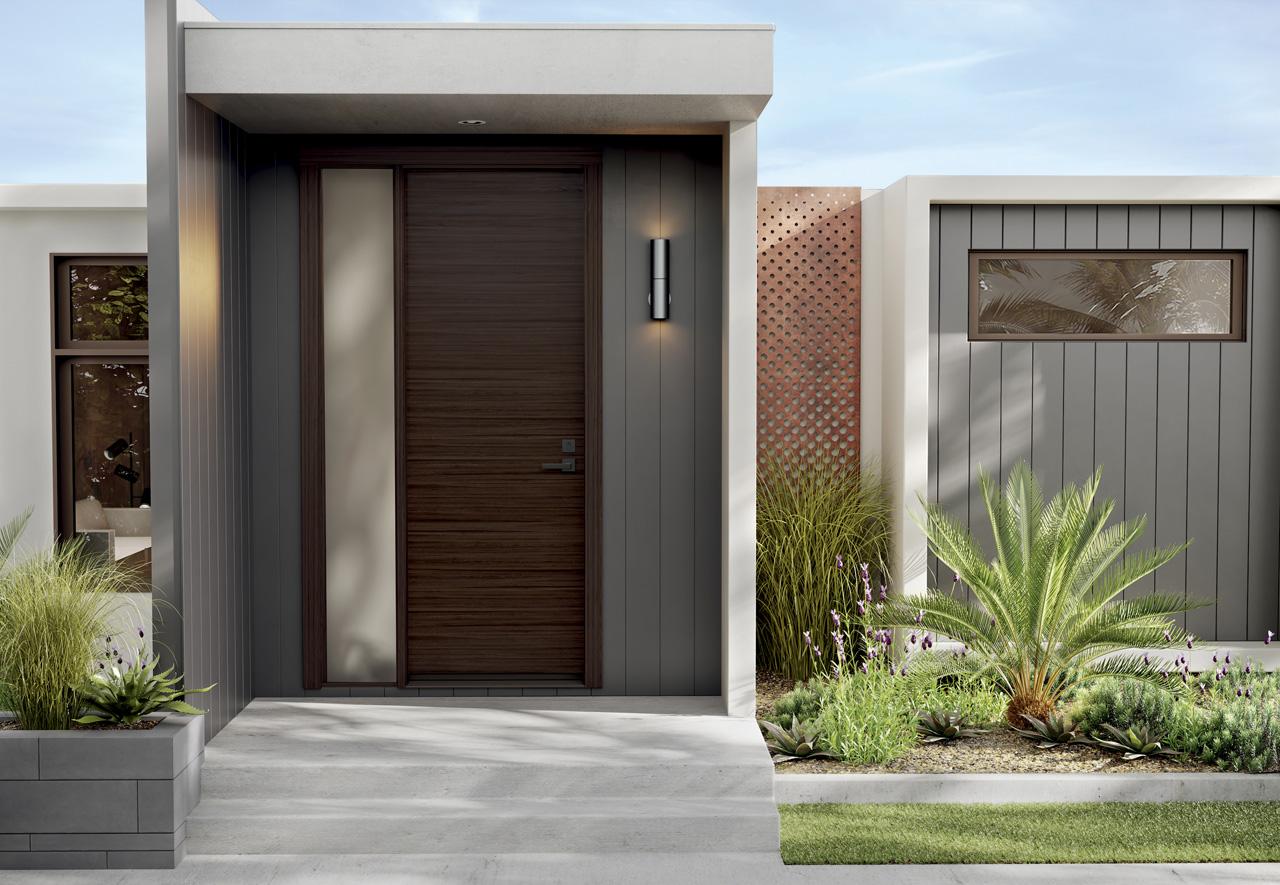This image showcases the front of a very modern, luxurious house, reminiscent of the mod-style homes you might find in Malibu or the west coast around Los Angeles. The house, which appears quite expensive, features a stunning combination of contemporary architectural elements including vertical wooden lattice, natural wood, concrete, and stainless steel. The exterior is mostly composed of gray shiplap wall panels, brown and white finishes, and a distinctive white trim. 

The focal point of the front is the elegant dark brown wooden door, highlighted by its horizontal wood grain and brushed metal hardware including a black keyhole and doorknob. Flanking the door to the left is a full-length, frosted white window, while to the right, there is a sleek silver light fixture that emits a warm orange glow from both the top and bottom. Surrounding the entrance area are neat gray concrete steps leading up to the door.

The house is enveloped in well-maintained, drought-resistant landscaping, suitable for its likely Californian setting. To the left of the doorway, there is a gray brick planter filled with succulents and grasses, while on the right, a low green lawn runs along a narrow strip, interspersed with bushes and shrubs. Above the entrance, there is a practical overhang to protect from rain, further emphasizing the thoughtful design elements of the house. The scene is set against a backdrop of a clear, light blue sky, enhancing the overall pristine and curated look of the residence.